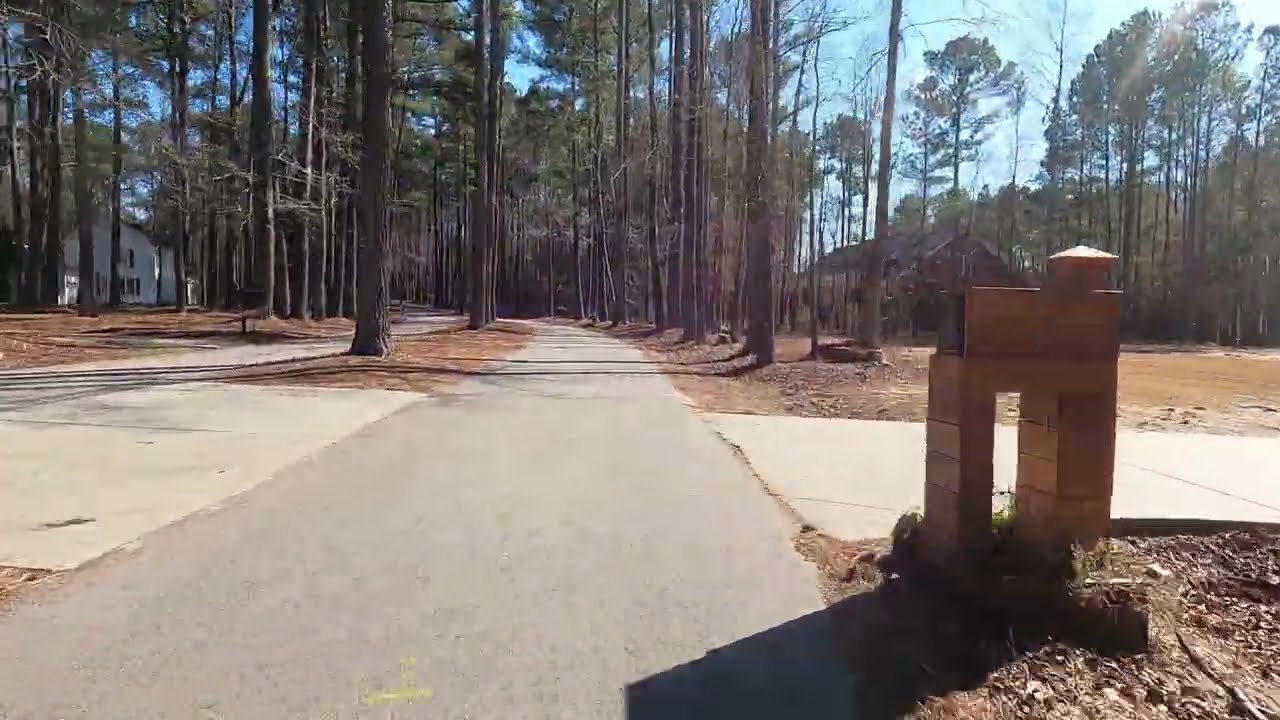The image depicts a serene, single-lane road that begins in the bottom left corner of the frame and continues towards the center before curving to the left. This road is divided by a grassy median with scattered tall trees. On the right side of the road, there's an elaborate brick mailbox marking the entrance to a driveway. This driveway leads to a dark, possibly brown, house nestled among the trees. On the left side of the road, there is a white house somewhat visible through the dense foliage. The background is filled with tall trees with green tops and brown trunks, casting shadows across the sunny scene. The clear blue sky above enhances the brightness of the day. Pine needles and leaves are scattered across the ground, adding to the natural and tranquil ambiance of this wooded neighborhood pathway.